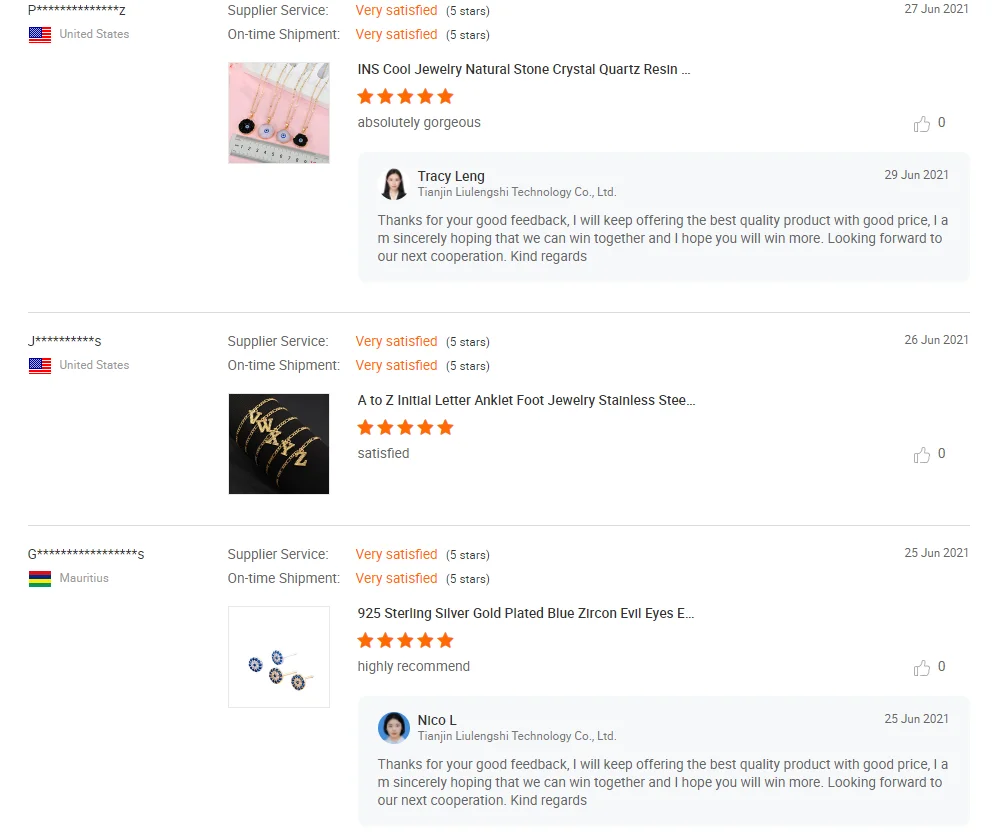The image depicts a detailed review section of a website featuring three separate reviews from various users. Each review is neatly divided by lines and reveals comprehensive feedback including ratings, text descriptions, and images of purchased jewelry.

**First Review:**
- **User:** P****Z
- **Country:** United States (indicated by the national flag)
- **Ratings:**
  - Supplier Service: Very Satisfied (5 stars)
  - On Time Shipment: Very Satisfied (5 stars)
- **Product Feedback:** Featured a photo of jewelry with the description:
  - **Product:** INS Cool Jewelry, Natural Crystal Quartz Resin
  - **Rating:** 5 stars
  - **Comment:** "Absolutely Gorgeous"
- **Additional Feedback:** Message from Tracy Lang thanking for the feedback and expressing hopes for continued cooperation.

**Second Review:**
- **User:** J****S
- **Country:** United States (indicated by the national flag)
- **Ratings:**
  - Supplier Service: Very Satisfied (5 stars)
  - On Time Shipment: Very Satisfied (5 stars)
- **Product Feedback:** Included an image of various jewelry items with the description:
  - **Product:** A to Z Initial, Letter Anklet, Foot Jewelry, Stainless Steel
  - **Rating:** Satisfied

**Third Review:**
- **User:** G****S
- **Country:** Mauritius (indicated by the national flag)
- **Ratings:**
  - Supplier Service: Very Satisfied (5 stars)
  - On Time Shipment: Very Satisfied (5 stars)
- **Product Feedback:** Displayed an image of earrings with the description:
  - **Product:** 925 Sterling Silver Gold-Plated with Blue Zircon, Evil Eyes
  - **Comment:** Highly Recommended
- **Additional Feedback:** Similar to the first review, a thank you message for the good feedback, with a promise of providing high-quality products at good prices and hopes for future successful cooperation.